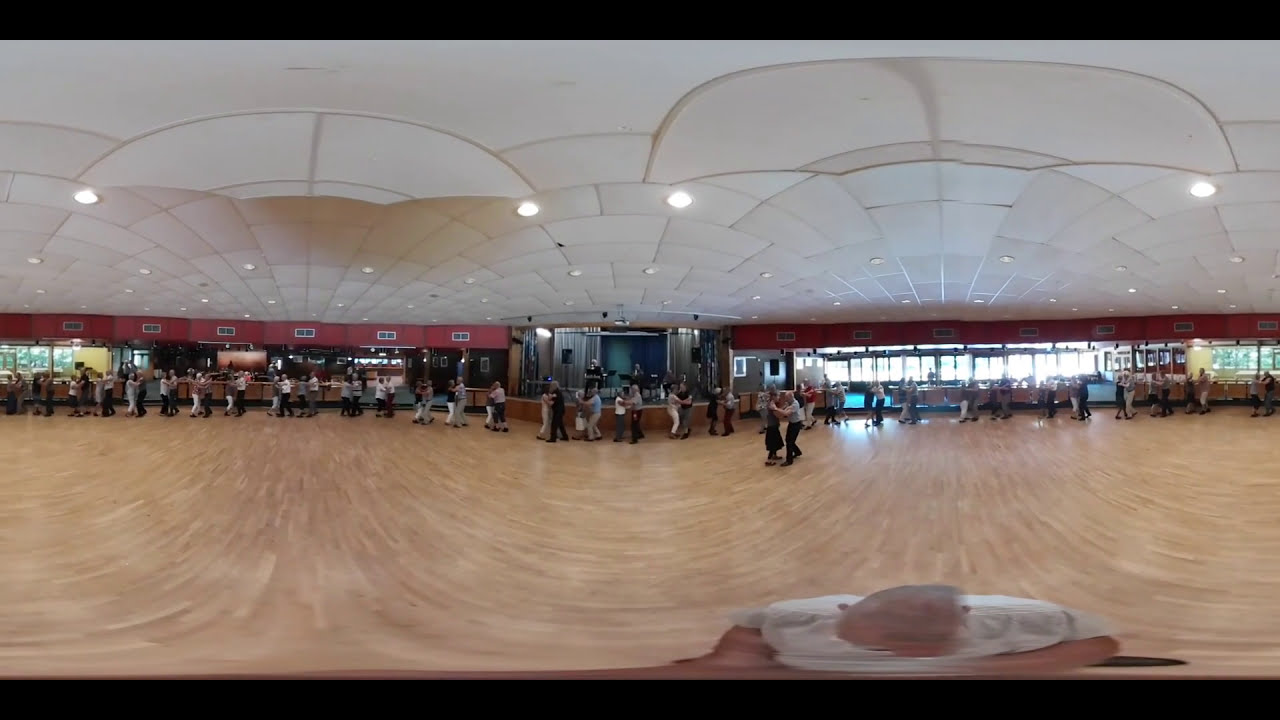This image captures a vibrant scene inside a well-lit dance hall, showcasing an elegant setting with red walls, a light brown wooden floor, and a detailed white ceiling adorned with lights. The photograph seems slightly distorted, likely due to it being a panoramic or 360-degree image, and features thin black bars at the top and bottom, resembling a still from a video. Approximately 30 elderly couples, most likely in their 70s to 90s and predominantly Caucasian, are seen dancing closely with each other, enjoying the lively atmosphere. At the center, a band performs on a stage backed by gray curtains and a blue backdrop, with music stands visible. The room also features large windows letting in ample daylight, enhancing the cheerful ambiance, and there appears to be a bar or restaurant area in the background. In the foreground, part of a person in a white shirt handling equipment is visible, adding to the dynamic, bustling energy of the scene.